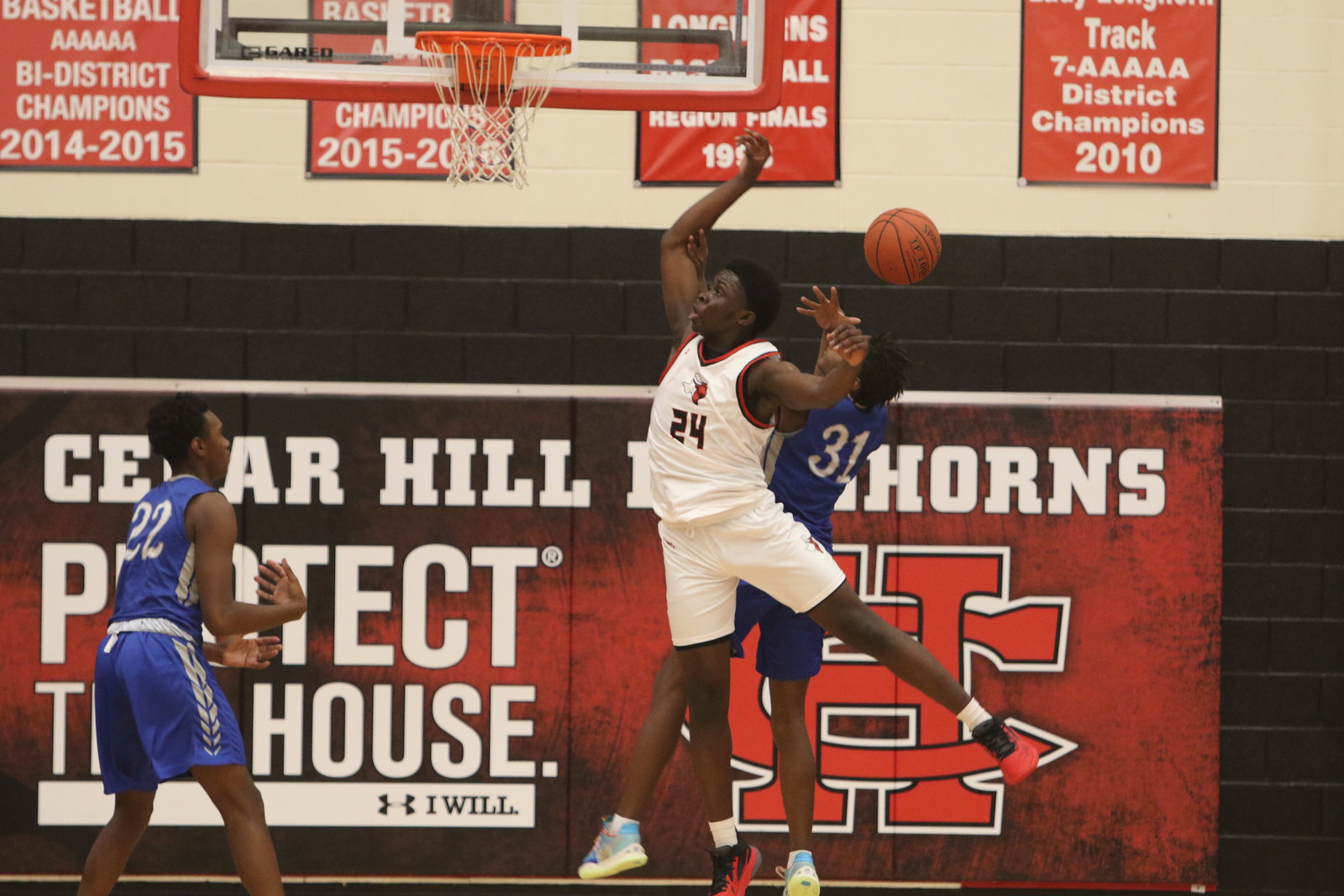The photo captures a high school basketball game in mid-action within a gymnasium adorned with championship banners. At the center of the frame, an African-American player is airborne trying to make a basket. He wears a white uniform with the number 24 emblazoned on his chest. As he aims for the hoop just left of center at the top of the image, the basketball is seen flying out of his hands due to an opposing player’s successful defensive move. This defensive player, also African-American and donning a blue uniform with the number 31 on his back, is positioned slightly behind and extending his hand to tap the ball away, touching 24's inner elbow. To the lower left, another African-American player in a blue uniform with the number 22 stands poised under the hoop, readying himself for the next move. The background wall is divided into a light tan upper section with red and white banners and a lower section of black cinder blocks. The banners detail various championships, including "Basketball District Champions 2014-2015" and "Track District Champions 2010." A prominent banner on the wall reads "Cedar Hill Protect the House," partially obscured by the players' dynamic presence in the foreground.